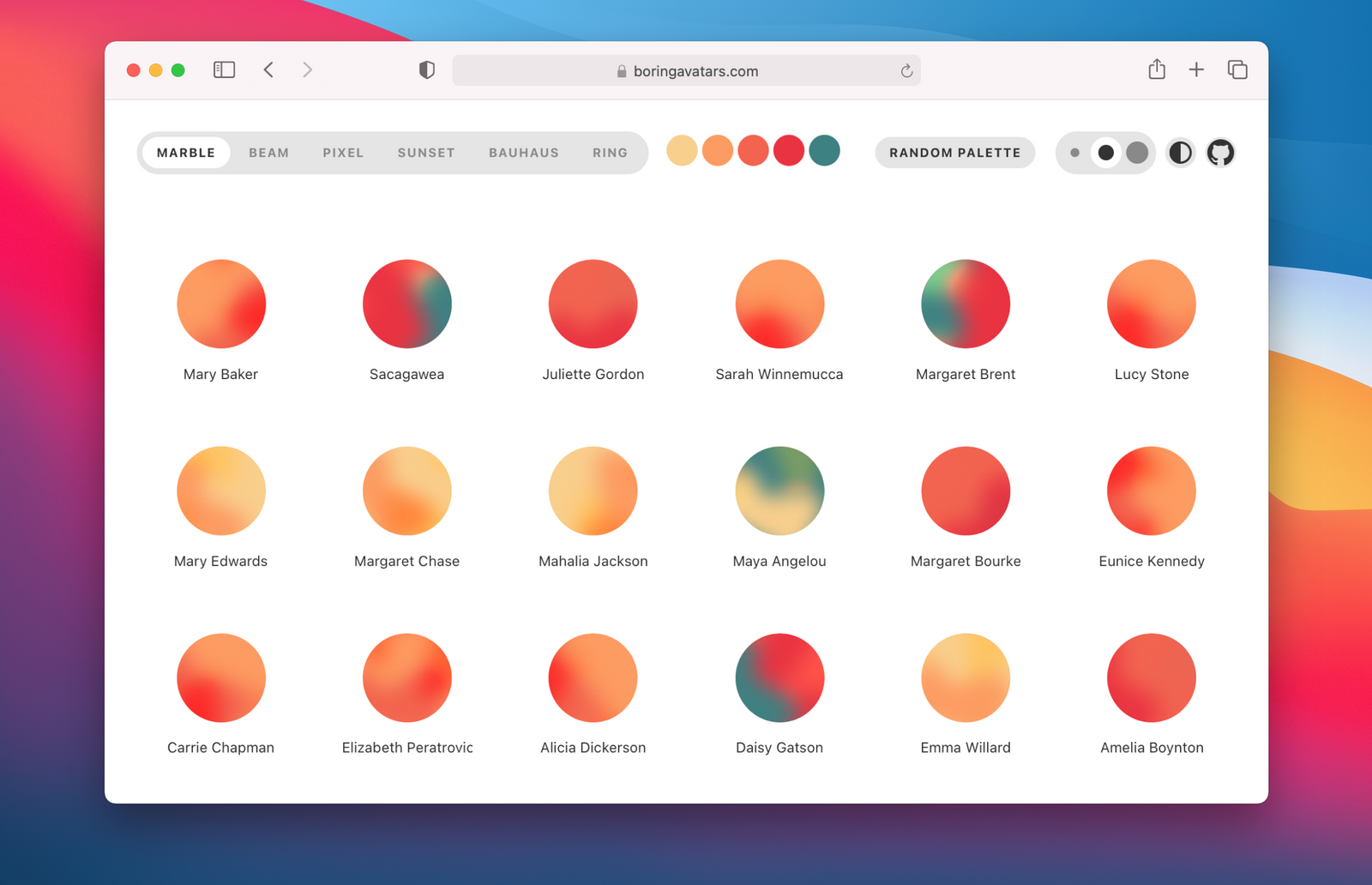The image features a visually dynamic and colorful composition with a variety of geometric shapes and hues. The background showcases a "Boring Avatars" design styled as a marble pattern, primarily highlighted in white and reminiscent of a pixelated sunset scene within a house. At the center, there is an arrangement of five circles in distinct colors: yellow, orange, pinkish-red, red, and blue.

Additionally, the composition includes various gray tones—a gray circle, a black circle, and a larger gray circle—forming a contrasting palette. There is also a circle that is half black and half white, positioned towards the right side of the image. One prominent element is a black circle displaying a cat icon.

Surrounding these central elements are numerous smaller circles, each labeled with specific names: 
1. Mary Baker 
2. Sacagawea 
3. Juliette Gordon 
4. Sarah Winnemucca 
5. Margaret Brent 
6. Lucy Stone 
7. Mary Edwards 
8. Margaret Chase 
9. Hala Jackson 
10. Maya Angelou 
11. Margaret Bourke-White

The diverse palette and structured layout create an eye-catching and meaningful artistic piece.